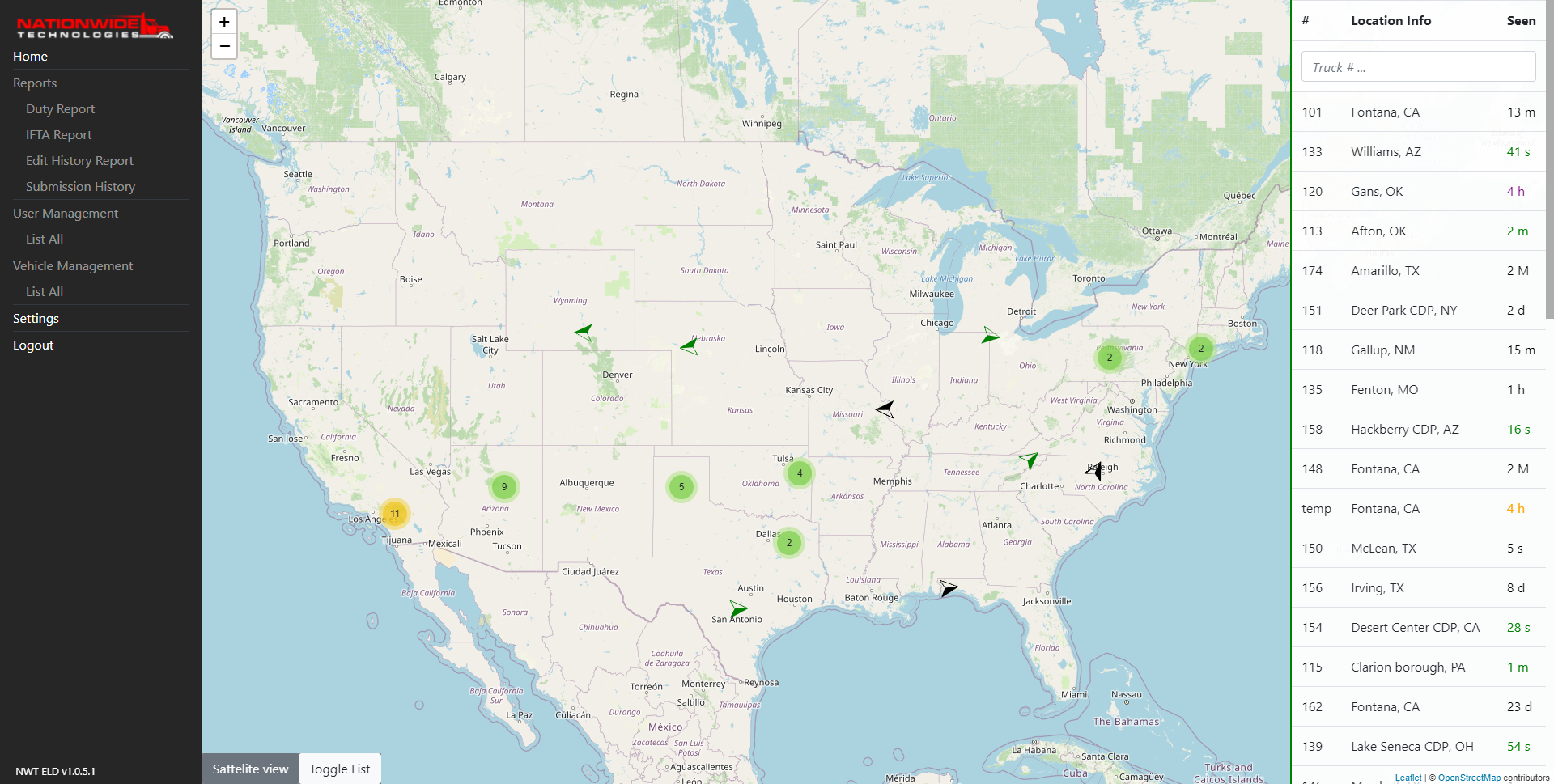Screenshot of Nationwide Technologies website, displaying the interface of their fleet management system. The main screen has a gray background with a red truck cab logo on the right side of the "Nationwide Technologies" text, although the design appears somewhat unconventional. On the left side, a vertical menu lists several options: Home, Reports, Duty Report, IFTA Report, History Report, Submission History, User Management, List All Vehicles, Management List All, Settings, and Logout.

The main panel features a map of the United States dotted with circles that include numbers, signifying various locations. Key points shown include:
- California (Yellow circle with a "11")
- Arizona (Yellow circle with an "8")
- Texas (Yellow circles with "2" and "5")
- Oklahoma (Yellow circle with a "4")

These markings likely represent active fleet or key site locations rather than sequential ordering. 

To the right of the map, there is a "Location Info" section detailing recent position reports for each truck including:
- Truck 101 in Fontana, California, last seen 12 minutes ago.
- Truck 133 in Williams, Arizona, last seen 41 seconds ago.
- Truck 120 in Gans, Oklahoma, last seen 4 hours ago.
- Truck 113 in Elton, Oklahoma, last seen 2 minutes ago.
- Truck 134 in Amarillo, Texas, last seen 2 minutes ago

This section continues with upwards of 20 entries, navigable via a scrollbar on the right. Additionally, there is a search bar for finding specific truck numbers. This detailed interface provides real-time tracking information for trucks operated by the company, showcasing the system's comprehensive fleet management capabilities.